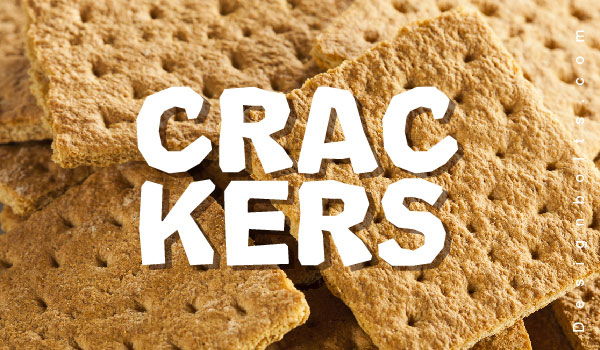This image appears to be an advertisement for crackers. It features a close-up shot of numerous dark brown, rectangular graham crackers with numerous small holes scattered across their surface. These crackers are piled together haphazardly, creating a textured background. In the center of the image, the word "CRACKERS" is prominently displayed in large, bold, white capital letters, split into two horizontal sections: "C-R-A-C" on the top line and "K-E-R-S" on the bottom line, giving the text a slight shadow effect. Additionally, in the corners of the image, specifically the right-hand side, there is a small, vertical watermark that reads "designbolts.com" in thin white text.